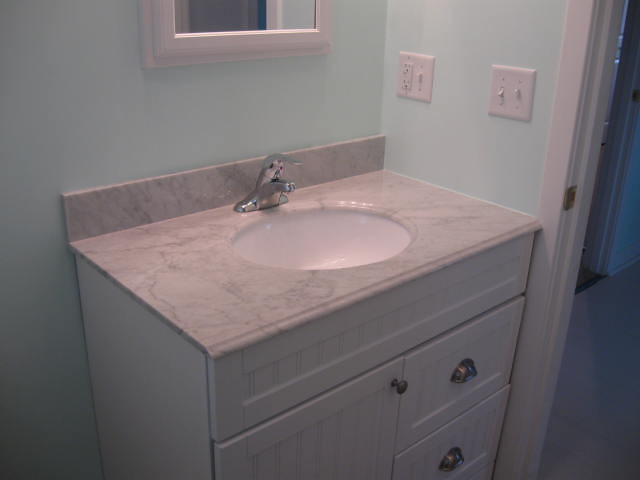This photograph showcases a bathroom with light green-colored walls. Dominating the scene is a mirror with a pink-painted wooden border on the outside. To the right of the mirror, there is an electrical outlet featuring two plugs and a switch, as well as another light switch with two toggles. Below these, the sink area is elegantly designed; it features a marble-like countertop with a subtle pinkish tint, supporting a white sink basin complete with a stainless steel faucet and handle. The sink is set into a white wooden cabinet that sports a tall door on the left side and two brass-handled drawers on the right. To the far right of the image, part of a door frame is visible, leading into a hallway where another door can be seen just a few feet beyond.